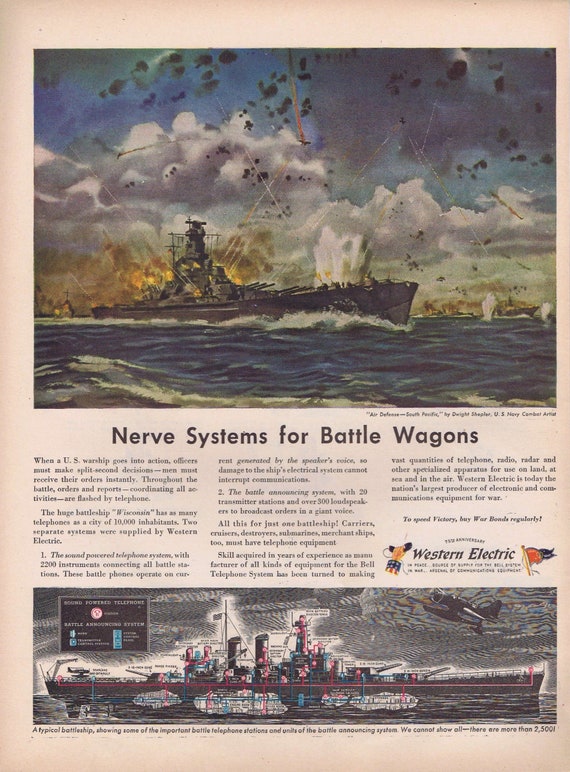The image appears to be a vintage magazine or newspaper cutout, possibly an advertisement or a news story, presented on an aged, beige-pink background. At the top, an illustration showcases a long black battleship sailing through choppy, blue waters with white waves. The sky above is filled with white clouds and gray smoke, indicating ongoing battle, with visible explosions, orange and yellow fire, and distant cannon fire. Amid this dramatic scene, a warplane with one propeller and multiple wings flies overhead. The title "Nerve Systems for Battle Wagons" is prominently displayed above the illustration.

Below this title, there are three columns of text formatted like a news article, explaining the importance of instant communication on U.S. warships during battle, detailing how orders and reports are flashed by telephone systems, crucial for coordinating activities under combat conditions. The text also mentions "Western Electric," the company likely responsible for these communication systems.

Beneath the text, another detailed illustration of the same battleship reveals its inner workings. This cross-sectional view highlights the ship's compartments and communication systems using red and blue lines, explained by a legend above. The ship is primarily shown in shades of gray, with the intricate network of red and blue pipes standing out. The illustration is meticulous, providing a glimpse into the technology that supports swift decision-making and coordination during naval engagements.